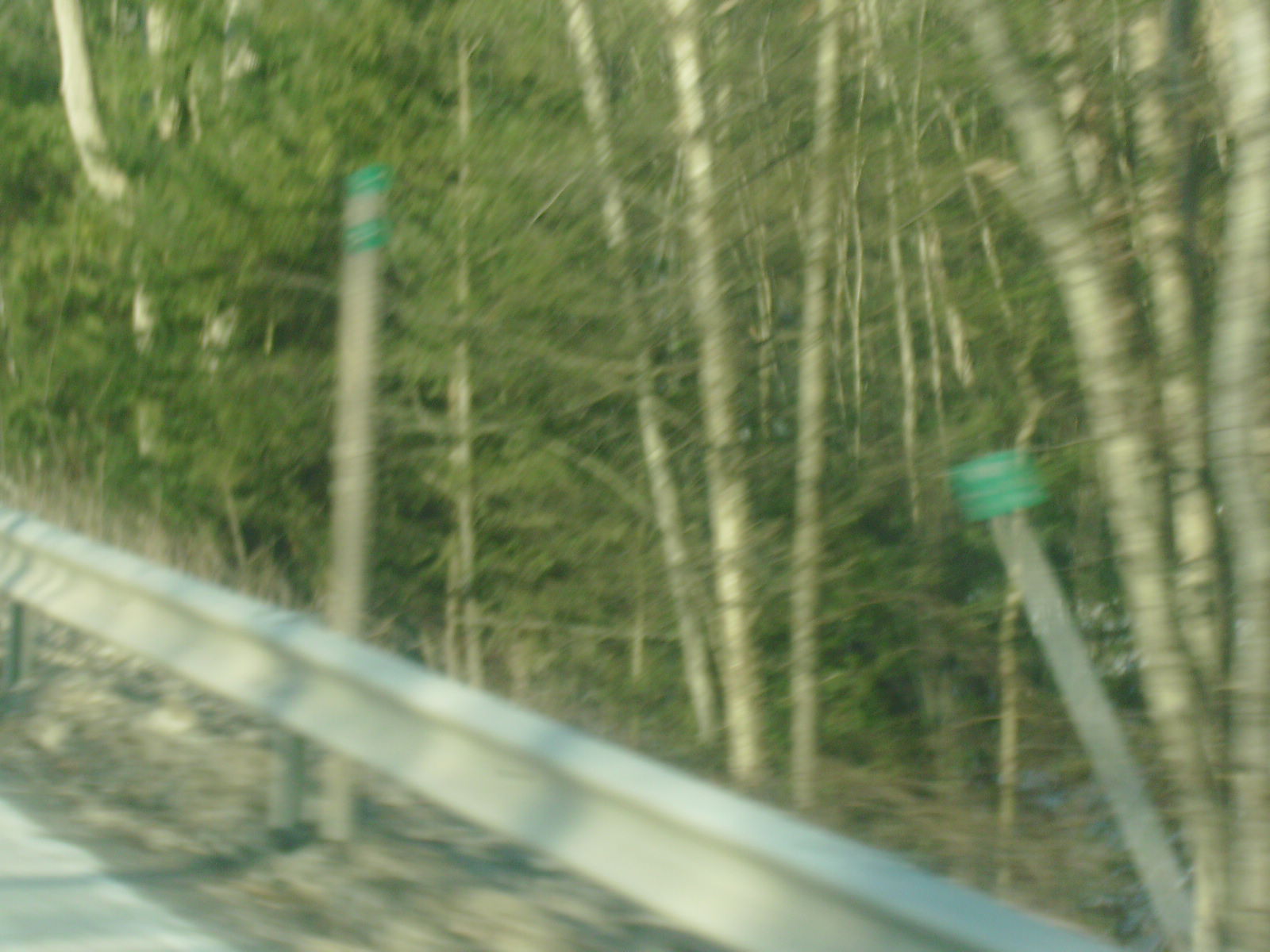A detailed caption for the image could be:

"The image captures the side of a road, partially visible in the bottom left corner. A guardrail runs diagonally across the bottom third of the picture, stretching from left to right. In front of the forest backdrop stand two poles, one of which is knocked over. Both poles feature green square signs, commonly used as mile markers. The background is densely packed with an array of slender, white-barked trees, resembling birch trees, adorned with lush green leaves. The scene is rich with a variety of branches weaving through the verdant forest, suggesting a road bordered by a thriving woodland."